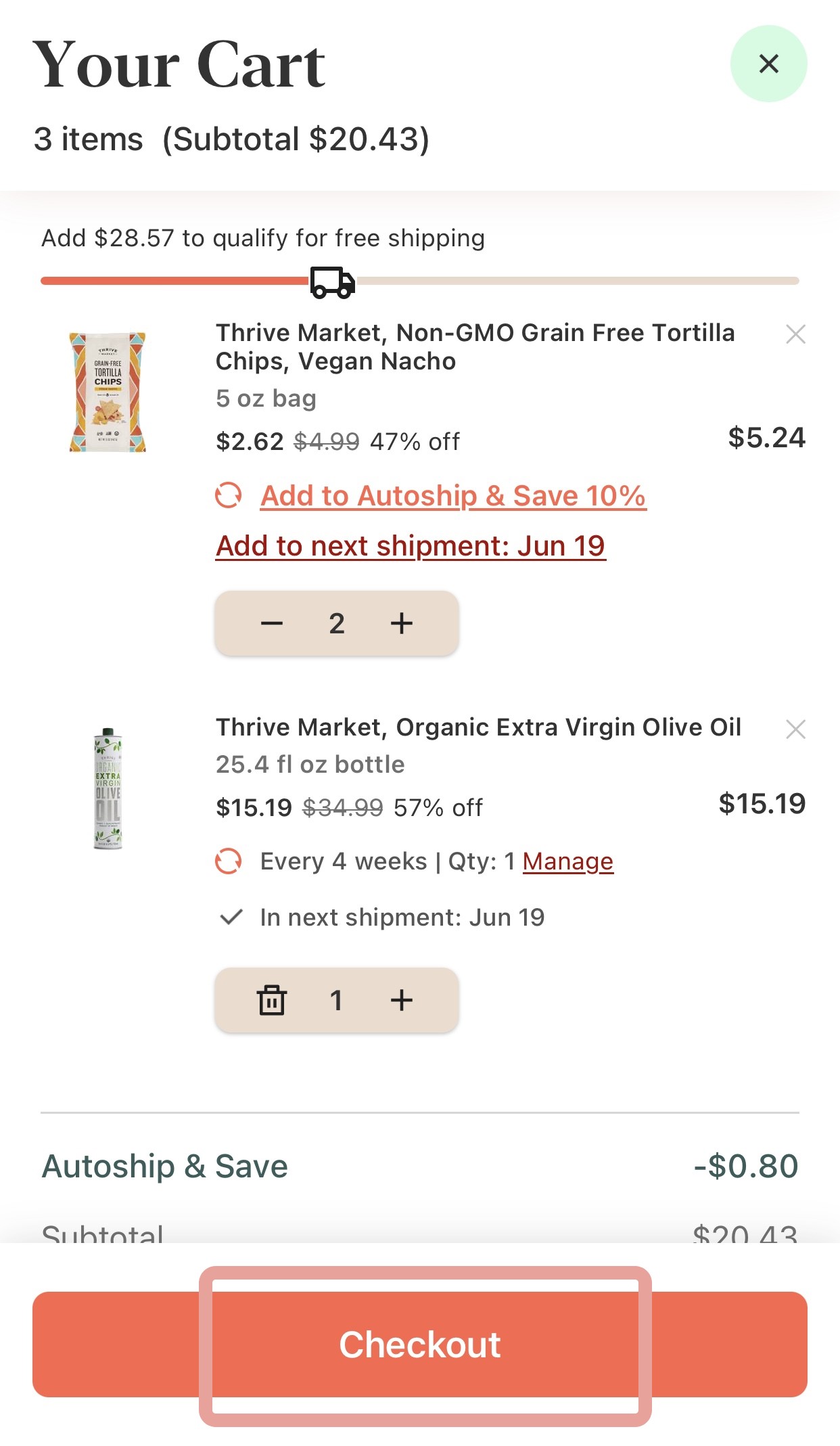The image depicts a shopping cart on an e-commerce website, likely focused on natural or organic products. At the top, bold black lettering states "Your Cart." The cart contains three items, with a subtotal of $20.43. A notification suggests that adding $28.57 more to the cart will qualify the order for free shipping, indicated by a small shipping truck icon.

The first item listed is two bags of Thrive Market Non-GMO Grain-Free Tortilla Chips in the Vegan Nacho flavor. Each 5-ounce bag is priced at $2.62, reflecting a 47% discount from the original $4.99 price, amounting to a total of $5.24. The product packaging is white adorned with a colorful southwestern pattern in blue, yellow, and red, evoking a desert aesthetic reminiscent of Arizona or New Mexico. There is an option to add this item to an auto-ship schedule, with the next shipment date being June 19th.

The second item is a 25.4 fluid ounce bottle of Thrive Market Organic Extra Virgin Olive Oil, priced at $15.19. It appears in a white bottle, presumably plastic rather than glass, consistent with the organic and sustainable shopping theme. This item is set to auto-ship every four weeks with a savings of 80 cents through the auto-ship program.

At the bottom of the cart, the subtotal is reiterated as $20.43. A prominent checkout button is displayed in a large, reddish hue, with the "Checkout" text highlighted by a pink rectangular outline.

Overall, the cart appears to be from a website specializing in organic and natural products, indicated by branding and item selection similar to retailers like Whole Foods.